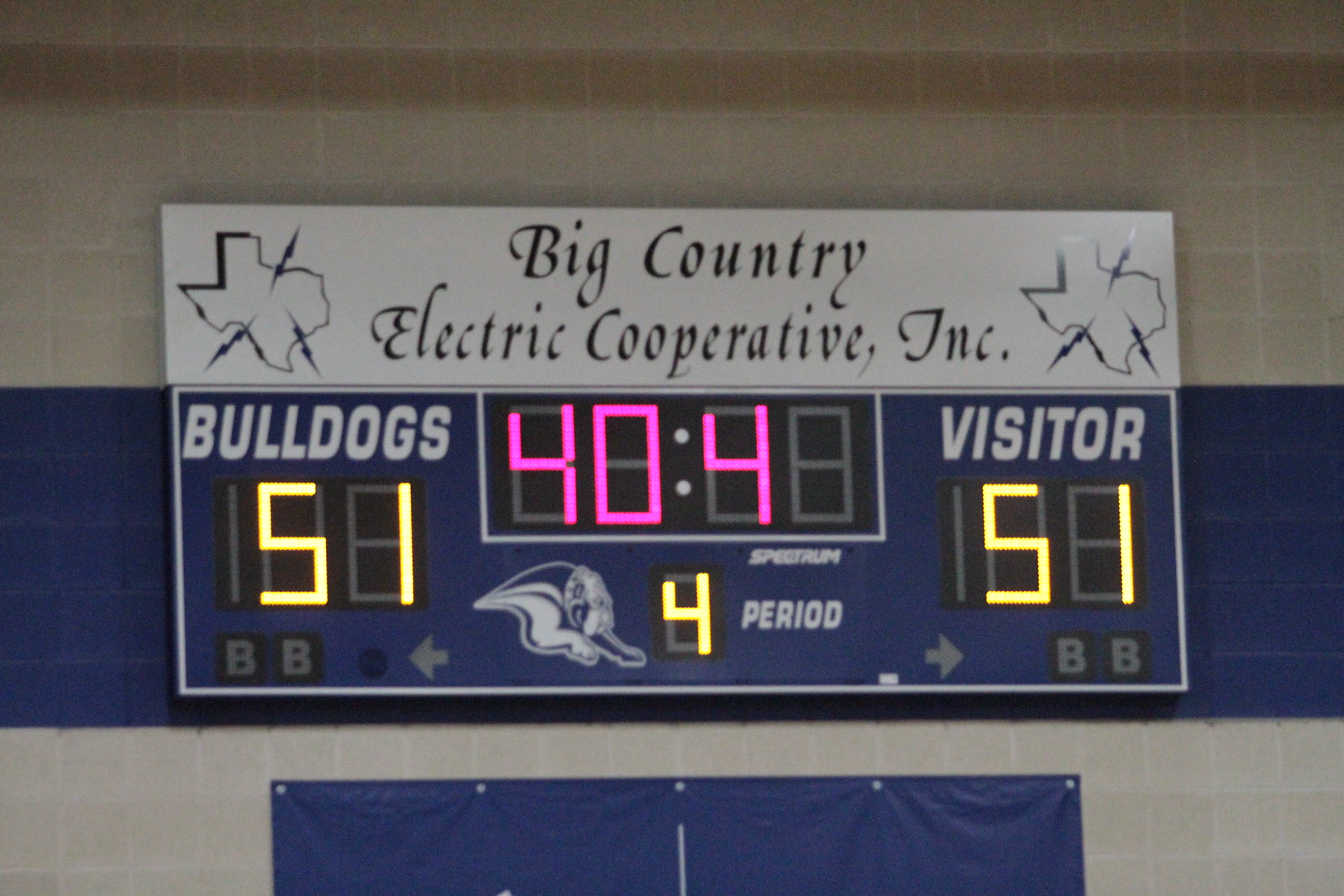This indoor photograph taken inside a gymnasium captures a digital scoreboard prominently fixed on a large wall. The rectangular image, wider than it is tall, displays the upper portion of the gym wall, which is brownish-gray with white grout, giving the impression of tiles. A significant feature of the wall is a wide blue stripe that stretches horizontally across just below the center. Directly beneath the stripe, a blue banner is pinned to the wall. The focal point of the photo is the scoreboard, marked at the top with "Big Country Electric Cooperative, Inc." and flanked by images of Texas with lightning bolts on each side, symbolizing the sponsor's logo.

The scoreboard details reveal a tense match, with "Bulldogs" and "Visitors" displayed on either side, both teams shown to be tied at 51 points. The current period is indicated as the fourth, with time left showing as 40.4 seconds. The scoreboard's background is predominantly gray and blue, with specific details in black, white, pink, and yellow, clarifying team names and scores. The lower portion of the wall again features the continuation of the blue stripe and just above it, a part of the blue banner is visible. The scene suggests a pivotal moment in a basketball game, with the highly detailed scoreboard providing a focal point against the gym's contrasting wall textures.